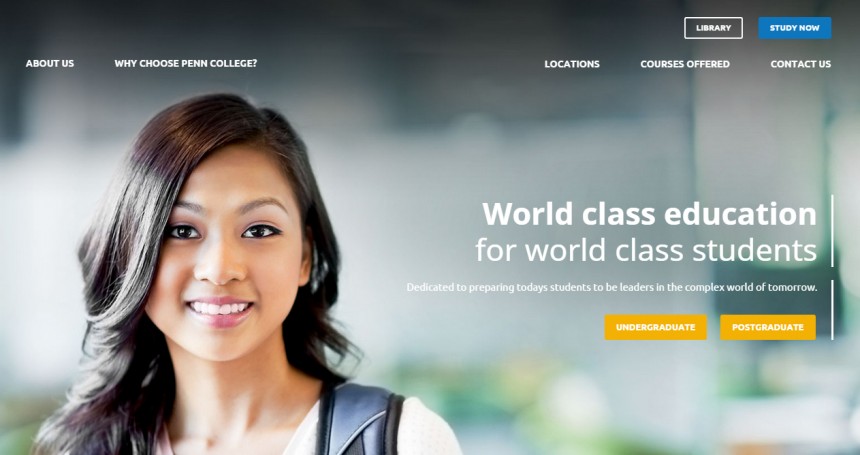This screenshot is from a Penn College webpage. The background features a very blurry image of what appears to be one of the college buildings. The image has a predominantly gray tone, with patches of green at the bottom, likely indicating shrubs or grass. On the left side of the image, there is an Asian girl who looks to be of college age. She is smiling at the camera and has dark hair with purple highlights, complemented by pink lipstick. She is wearing a white V-neck shirt, visible down to just below her neckline, and is carrying a gray backpack.

In the upper right corner, there is a white box with text in white letters that reads "Library," next to a blue box with white text that says "Study Now." Below these boxes are additional options in white text, including "About Us," "Why Choose Penn College?," "Locations," "Courses Offered," and "Contact Us." The text continues with the phrases "World-class education for world-class students" and "Dedicated to preparing today's students to be leaders in the complex world of tomorrow," both written in white.

At the bottom of the image, there are two orange or gold rectangular boxes. The box on the left has white lettering that reads "Undergraduate," while the box on the right also has white lettering and reads "Post-graduate."